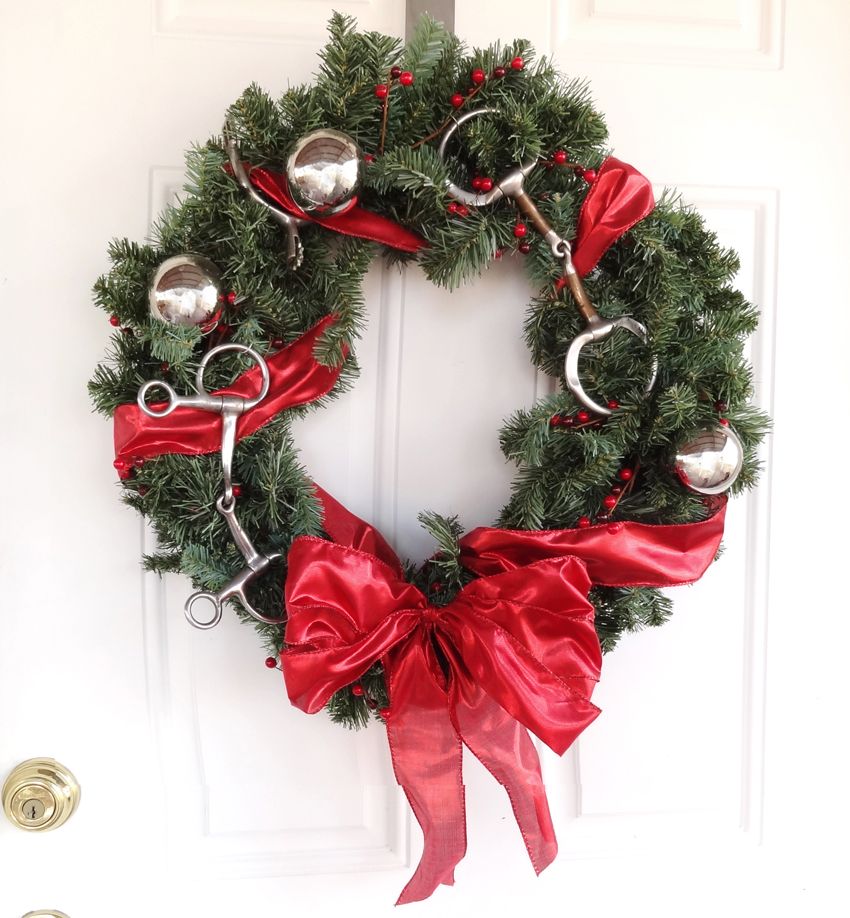This photograph captures a festive Christmas wreath hanging on a white door, which features a gold key insert. The dark green wreath is adorned with an array of holiday decorations, including red ribbon that wraps around it and culminates in a red bow at the bottom. Scattered throughout are clusters of fake red berries, adding a pop of color. The wreath also boasts several large, spherical silver ornaments that shimmer against the green. An unusual detail includes two metal pieces—one resembling the handle of scissors linked by additional metal parts, and the other akin to a set of handcuffs—woven into the wreath, creating a curious contrast to the traditional holiday elements. The wreath is securely hung by a silver hook over the top of the door.